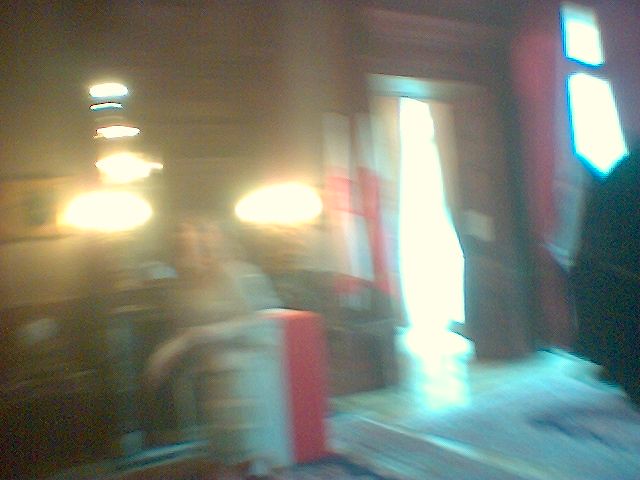A blurred image depicts the interior of an ambiguous building, possibly a public or private space but likely not a house. The design of the doorway, which is relatively large, suggests a non-residential structure. Sunlight pours through the entryway, illuminating the scene. Positioned on the left side of the image is a person clad in what appears to be a checkered dress, suggesting a female figure. Above and around the person's head are two large lights, adding brightness to the area. Adjacent to the bright light is a long red curtain through which additional light filters. The floor appears to be made of marble, partially covered by an area rug.